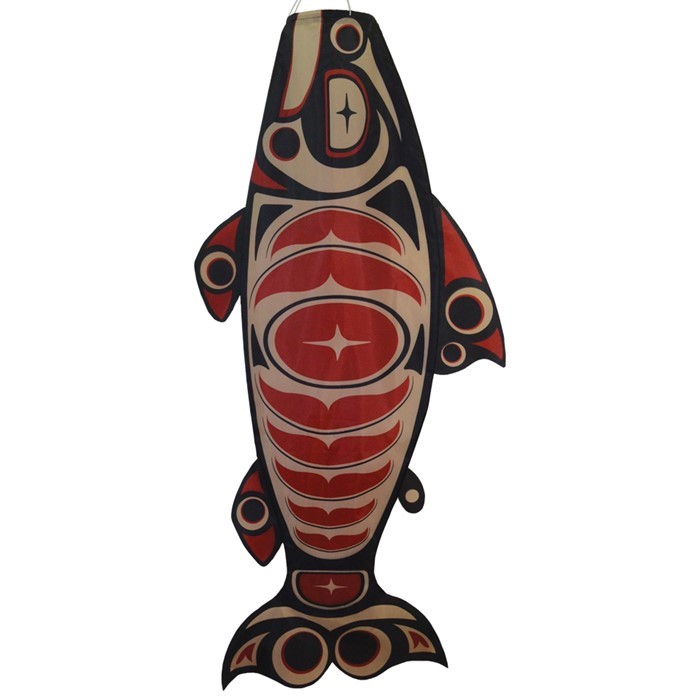The image depicts a vertically oriented, intricately carved wooden fish sculpture with its head pointing upwards and tail downwards, set against a solid white background. The fish is decorated in a distinctive Alaskan Indigenous art style, characterized by bold geometric shapes and vibrant color patterns. The sculpture is predominantly black, red, and tan, with extensive use of circular holes resembling eyes on the fins: two on the top fin, one on each bottom fin, and two on the back fin. These holes are accented in tan, red, and black. The fish's body is detailed with red bow-shaped designs and a large central oval with a star-like pattern in beige. The entire design is outlined in black, giving it a stylized and striking appearance. The fish's face is beige with red and black detailing, adding a further layer of intricate design. This decorative piece, possibly a wall hanging or a kite, evokes the style of North American Indigenous tribes, particularly reminiscent of those from Alaska known for their totemic art.